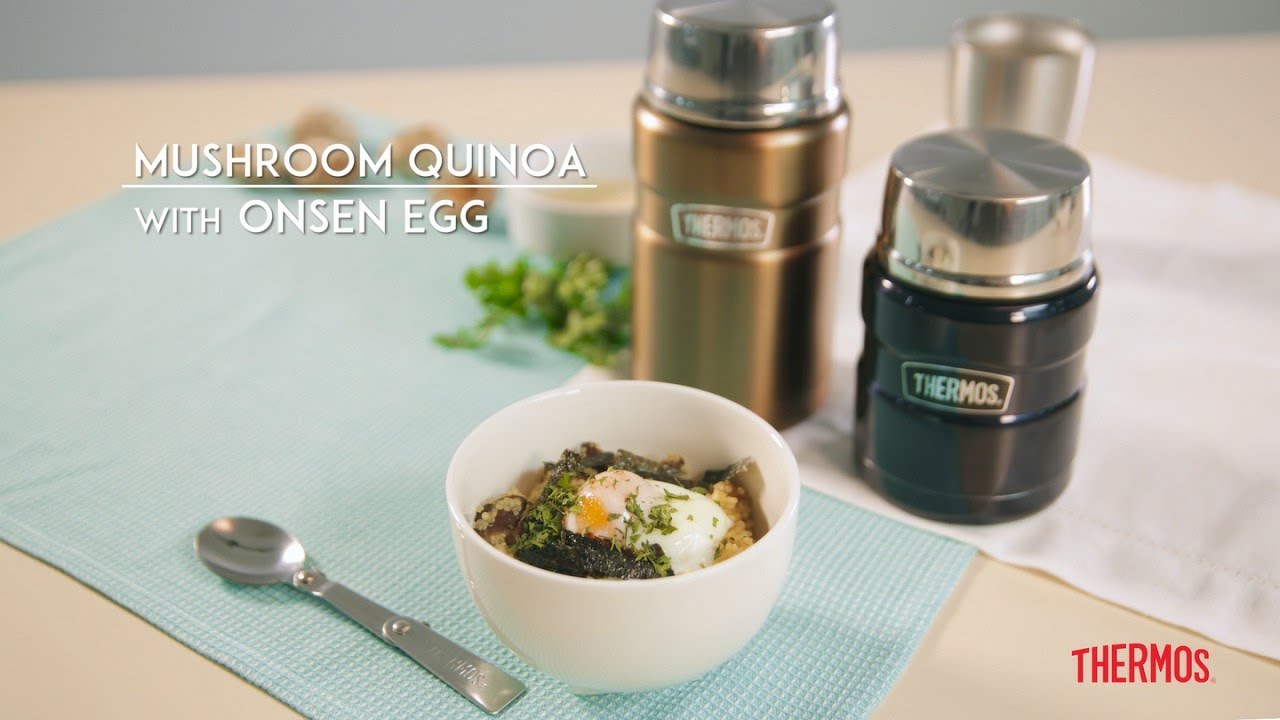The image is a horizontal, rectangular advertisement showcasing two Thermos products on a light-colored table, which appears to be beige or light wood. Toward the right side of the image, there are two thermoses—a shorter brown one and a taller black one—each with stainless steel lids and the brand "Thermos" displayed on them. Partially visible behind these is the metal top of a third item, possibly another thermos or a salt or pepper shaker, cut off by the edge of the frame. These thermoses are stationed on a white placemat. 

In the foreground, on a blue placemat, sits a white bowl containing a sunny side up egg, some greens, and brownish food items, likely mushroom quinoa with seasoning, accompanied by a silver spoon placed to the right of the bowl. The table setting is lightened by ambient beige tones, creating a minimalist and clean look.

The background of the image is also beige, with white lettering in the top left corner that reads "mushroom quinoa with onsen egg." The bottom right corner features the Thermos logo in red font, reinforcing the branded nature of the advertisement. The clean, organized layout combined with the clear depiction of the food and thermoses emphasizes Thermos' role in keeping your food warm and fresh.